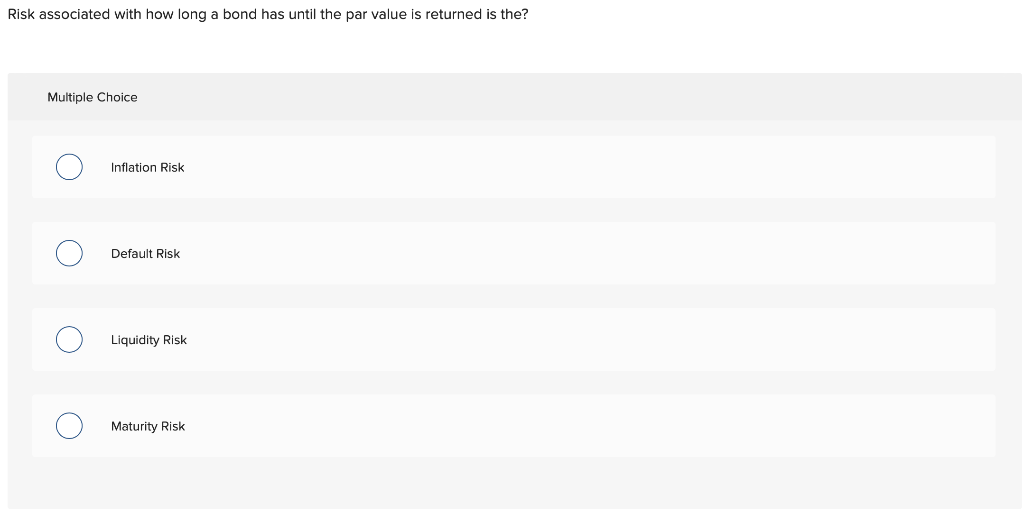The image depicts an online quiz or test focusing on financial concepts. At the top-left corner, the title reads, "Risk associated with how long a bond has until a par value is returned is the...?" Below this incomplete statement, there's a large grey box indicating the multiple-choice format of the question. The quiz presents four answer options, each preceded by a small blue circle. The options are: 
1. Inflation risk
2. Default risk
3. Liquidity risk
4. Maturity risk 

The layout suggests an interactive element where users can select their answer.